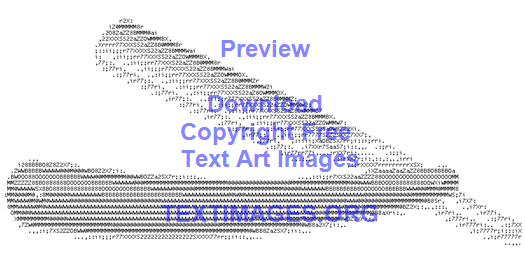The image is a detailed black-and-white text art graphic depicting a vintage barber's straight razor against a white background. The razor, characterized by its long, hinged blade that folds into the handle, is meticulously created using various sizes and shades of gray text characters, reminiscent of old dot matrix printer art. The shading effectively highlights the blade's lighter tone and the handle's darker areas. Overlaying the center of the graphic in purple text is the message: "Preview, Download copyright free text art images, textimages.org." The precision of the text characters showcases the potential of creating intricate images solely through letters and numbers.